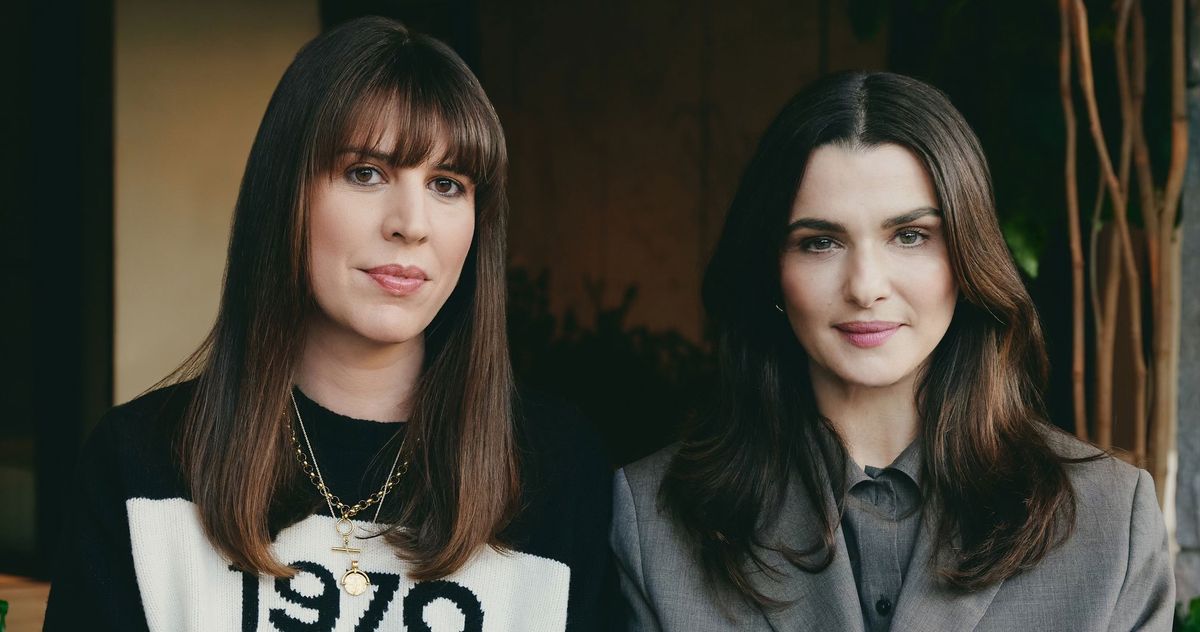The high-quality photograph captures two women, Rachel Weiss and Alice Birch, looking directly at the camera with detailed expressions and stylish outfits. On the left stands Rachel Weiss, distinguished by her straight brunette hair with long bangs framing her orange eyes and thick red lips. She wears a black sweater adorned with a white emblem displaying the year 1970, though the last digit is partly obscured. Her accessories include two gold necklaces, one with a medallion and the other a link-chain style. To her right is Alice Birch, characterized by her wavy brunette hair parted at the center, piercing brown eyes beneath thick eyebrows, and pink lips. She wears a black blazer over a gray, collared button-up shirt. The backdrop hints at an indoor setting, possibly a living room or office, featuring wood paneling and a small series of vines growing on the right side of the image.